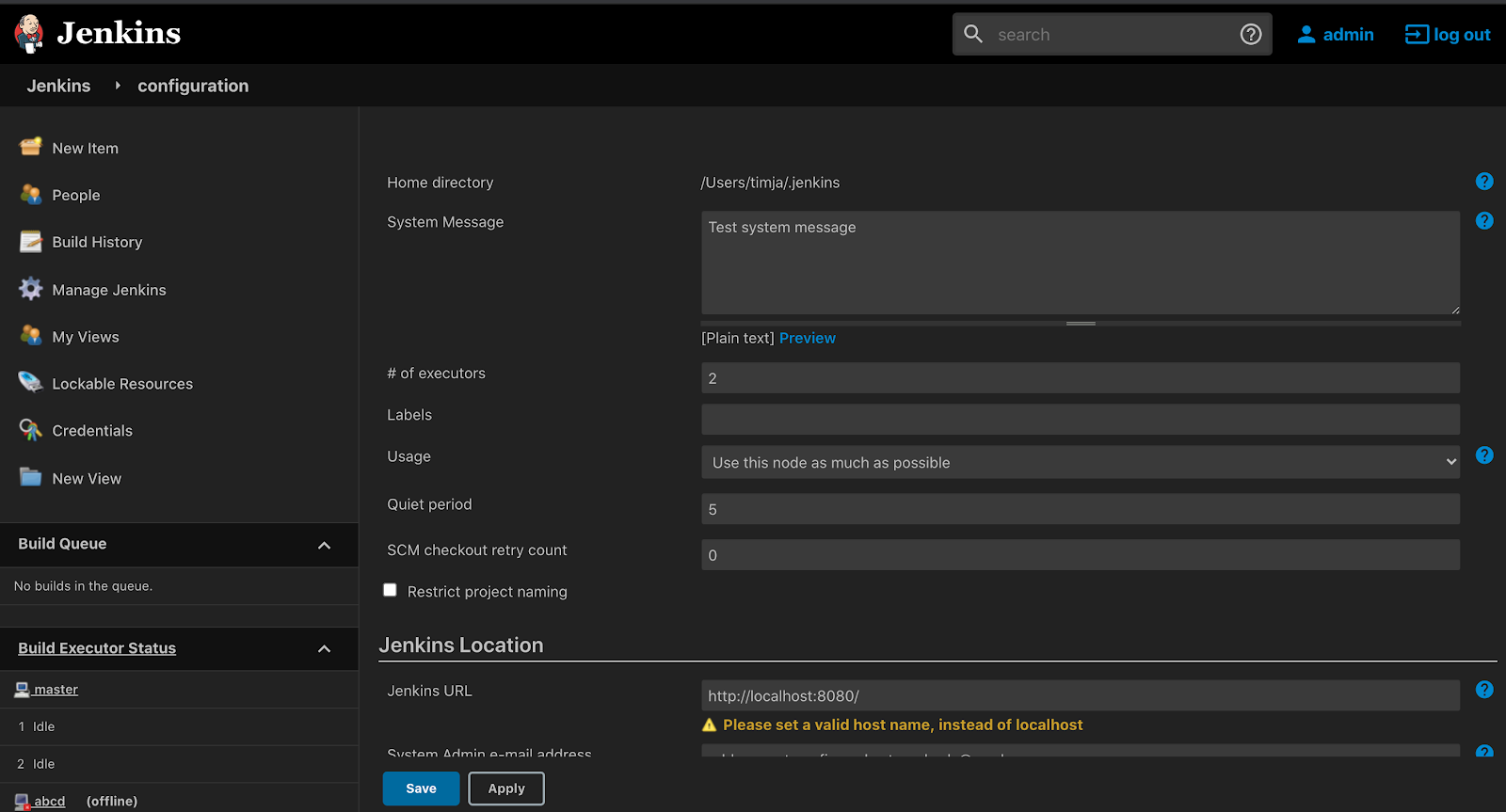The screenshot captures a Jenkins dashboard interface on a computer screen. The background is black, with white text detailing various sections and options. At the top, "Jenkins" is prominently displayed along with an illustration of a cartoon character. The navigation menu includes several options: "New Item," "People," "Build History," "Manage Jenkins," "My Views," "Lockable Resources," "Credentials," "New View," "Build Queue," and "Build Executor Status."

In the "Build Executor Status" area, it shows that "master," "one," and "two" executors are labeled as "killed," while "three ABC" is labeled as "offline."

Below, another section, headed with "search" and flanked by "administration" and "log out" in blue, shows details such as "home directory," specifically directing to "users/T-I-M-I-A Jenkins." A "system message" box, shown in gray, contains the text "test message system."

Further details include:
- Number of executors: 2 (in a gray box)
- Labels: an empty gray box
- Usage: "use this mode as much as possible" (in a gray box)
- Quiet period: 5 (in a gray box)
- SCM checkout retry count: 0 (in a gray box)
- Restrict project naming: checked

The "Jenkins Location" section contains inputs for "Jenkins URL," showing "http://localhost:8080." Below this, a highlighted note in orange suggests, "Please set a valid host name instead of localhost."

At the bottom, a "Save" button is present. The screenshot thoroughly captures the informational and navigational aspects of the Jenkins dashboard.